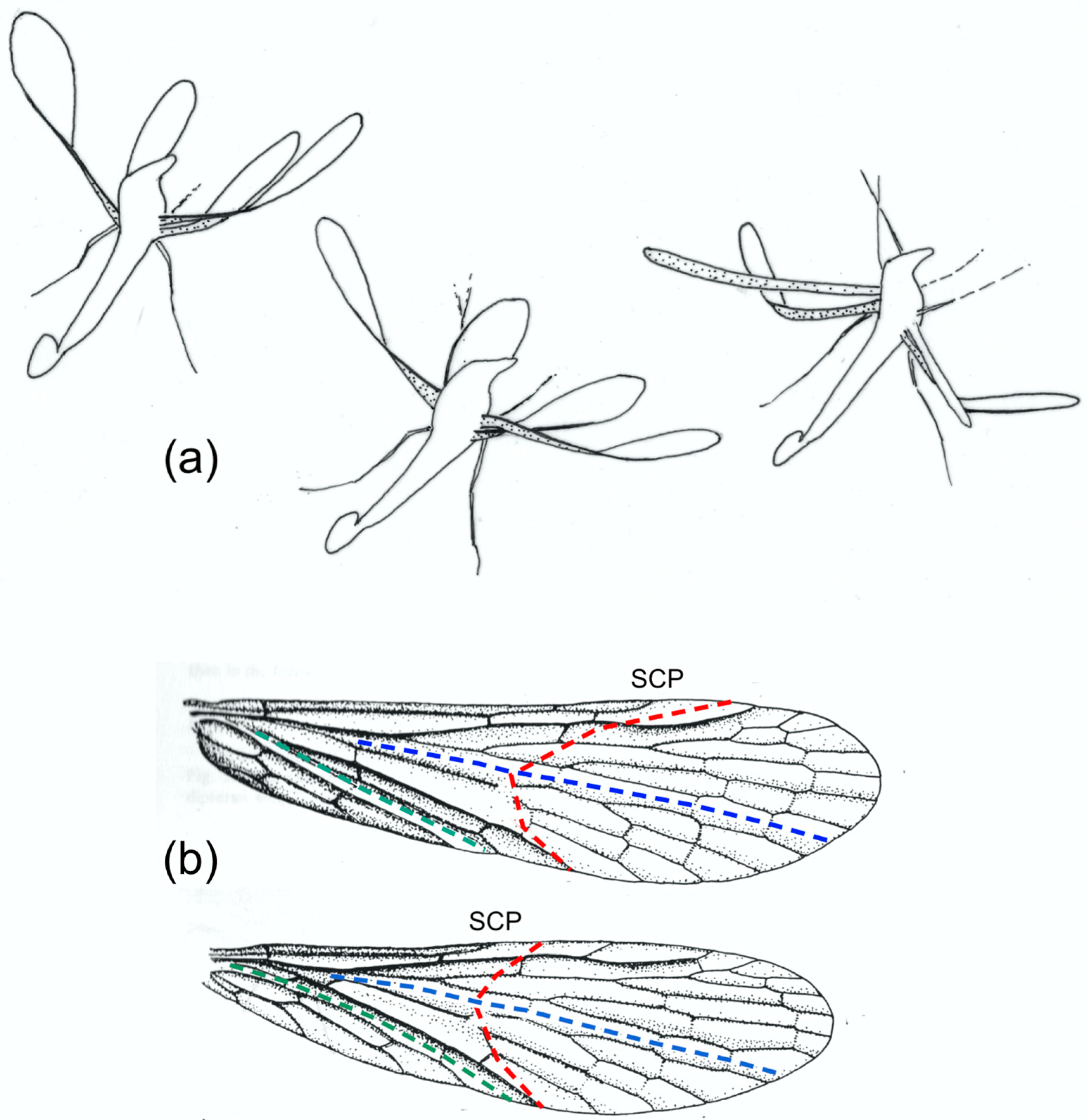The image is a black and white diagram divided into two sections, labeled A and B with parentheses in black text. In section A, at the top, there are three crude, basic line drawings of an insect resembling a dragonfly or moth. These insects are depicted with varying numbers of legs: six in the right drawing, four in the center, and three in the left. The drawings are simplistic and lack detail, depicting four wings, a long neck-like body, and a small abdomen.

In section B, at the bottom, there are two detailed artistic renditions of insect wings, also labeled SCP in large capital letters at the top of each wing. The wings have intricate patterns resembling cells or panels, with blue dotted lines running down the median and red dotted lines sectioning off areas. Additionally, green dotted lines are visible. The A wing has a larger area outlined in red compared to the B wing, and the wings collectively form an oval shape when viewed together.

The entire diagram is set against a white background, emphasizing the contrast and separation between the sections and the detailed and less detailed areas.